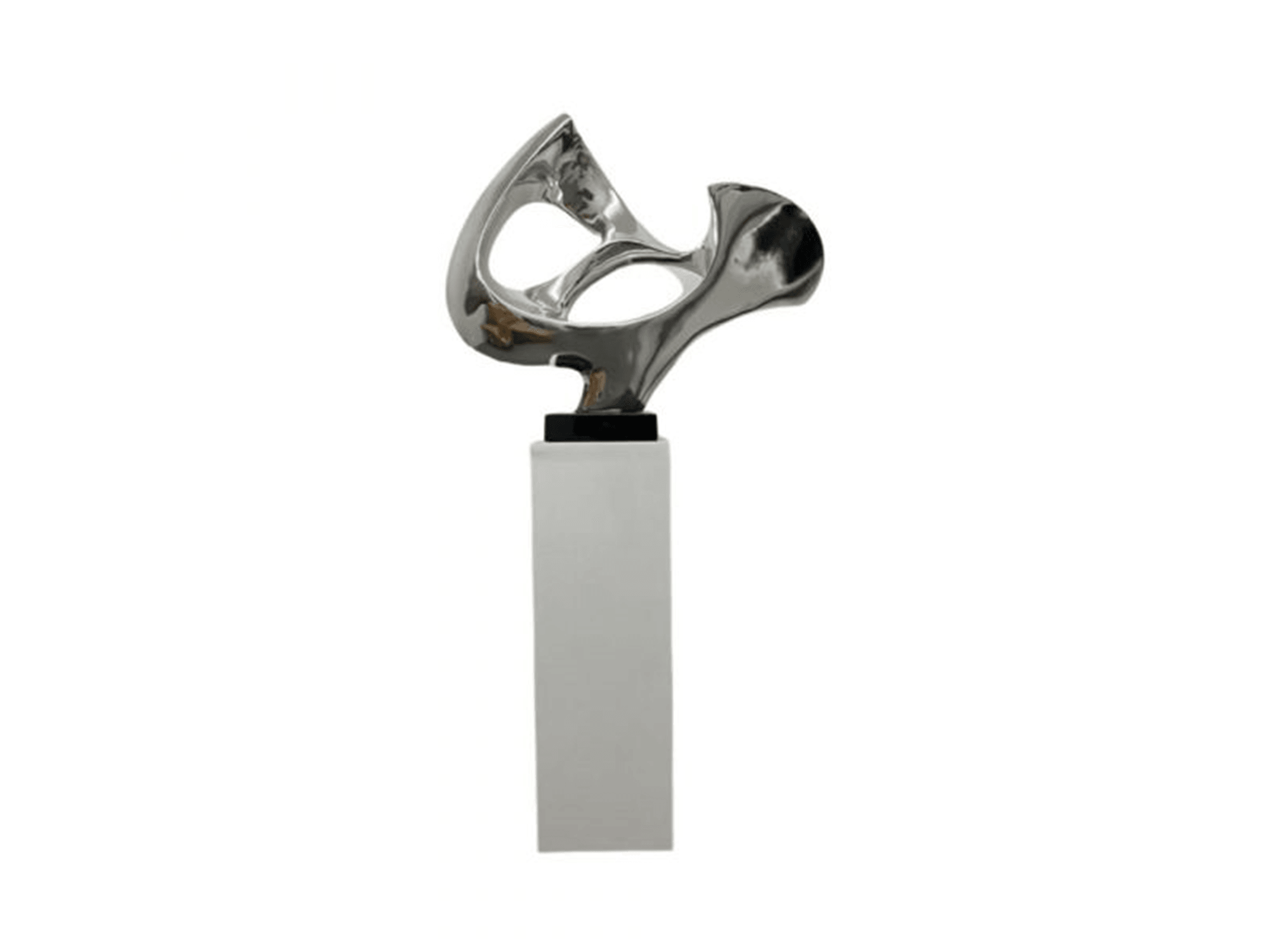The image features a modern art sculpture set against a pristine white background. The sculpture is mounted atop a tall, stone white pillar, enhanced by a narrow black rectangular pedestal approximately one inch thick. The piece itself is composed of a shiny, reflective metal, likely pewter or stainless steel, giving it a chrome-like finish. The design of the sculpture is random and geometric, characterized by varying thicknesses that create a dynamic and curving semicircle. The sculpture includes a structural element resembling a handle that arches across its center, contributing to its intricate form. The overall shape can be likened to a stylized 'U' with an extruded scoop and a central stripe of arcing metal, evoking the idea of a Möbius strip or a horseshoe, merging art and abstract geometry seamlessly.